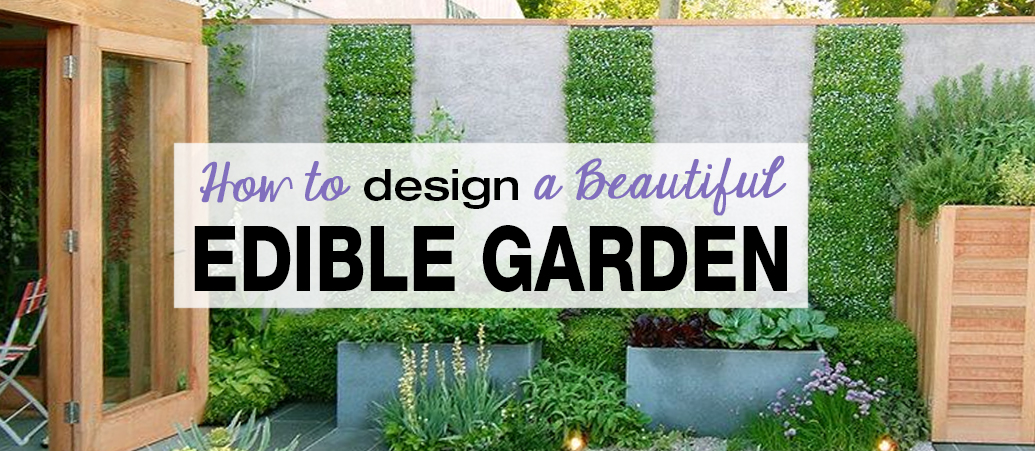In this photograph, a vibrant garden scene graces the background while bold text overlays the center, reading "How to Design a Beautiful Edible Garden." The phrase "how to" and "a beautiful" are written in elegant purple cursive, while the words "design" and "edible garden" are presented in sleek black sans serif, with the latter in thick, bold letters. The text is framed by a translucent white rectangle.

The garden consists of a cement wall occupying the upper half of the image, featuring three neatly trimmed, vivid green vertical strips of ivy climbing it. Below the wall, there are two cement planters— the left one showcasing green plants, and the right one containing green plants on its right and red-leafed plants on its left. A tall, unstained wooden planter brimming with bushy green plants stands to the wall’s right. To the left of the wall is an unstained wooden frame with an open door that has silver hinges and a central glass panel; behind this door is a similar window design. Inside the open door is a beach-style chair. The ground appears to be covered with shiny tiles, and a small portion of a house and some trees are visible above the wall along with more plants scattered around, enhancing the lush, outdoor aesthetic.